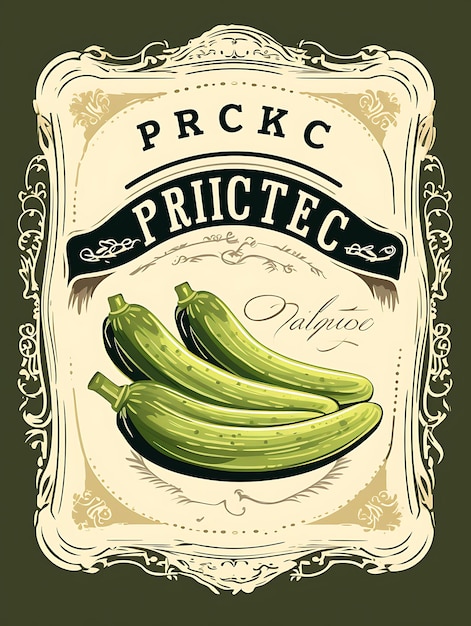The image features an advertisement, potentially from an old-fashioned postcard, showcasing three light green pickles or cucumbers. The background is olive green, with a white foreground where the vegetables are displayed. At the top, bold navy letters spell out "PRCKC," while a prominent beige banner in the middle reads "PRIICTEC," suggesting it might mean pickles or something related. Below this banner, there is ornate cursive text that is hard to decipher, potentially reading "NORTALQUOC." The overall design attempts to evoke a vintage feel, reminiscent of old-fashioned advertisements or vision test charts.